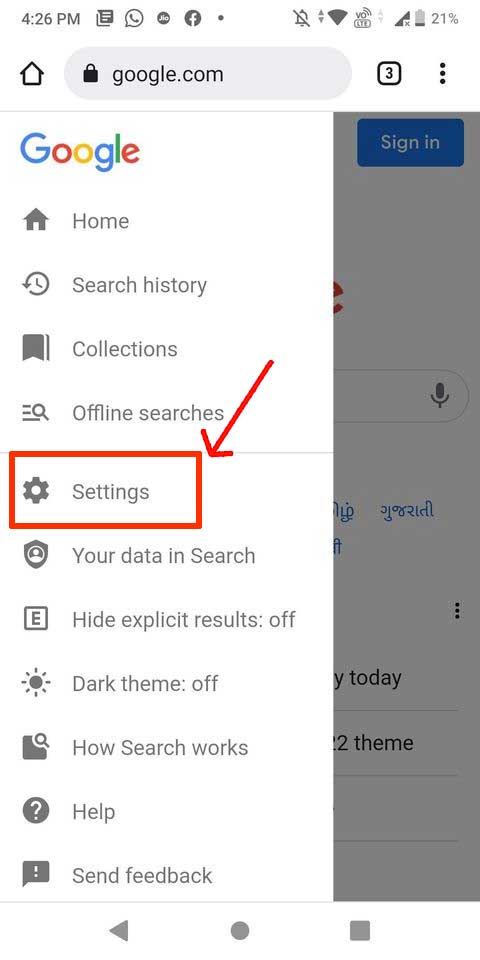The image showcases a smartphone screen actively accessing the Internet, with a header displaying the time as 4:26. The top section includes various icons: a phone call bubble, one for Facebook, and a bell with a line through it indicating the phone is set to silent mode. The battery level is shown at 21%.

The central part of the screen displays a web browser open to Google, with "Google.com" visible in the search bar, and a numeral "3" indicating the number of open tabs. Below the search bar is the Google homepage layout, featuring links to "Home," "Search History," "Collections," and "Offline Searches." A prominent red rectangle outlines the word "Settings," and a red arrow directs attention to this rectangle. Under the "Settings" section, the screen shows "Your Data in Search."

Further down, there's an "E" in a small box and options for "Hide Explicit Results" and "Dark Theme," both toggled off. Following these options are text links for "How Search Works" and a help section denoted by a bubble with a question mark, labeled "Help." Underneath is an option to "Send Feedback."

At the bottom of the screen, there is a navigation arrow pointing to the left, an oval-shaped button in the center, and a square button on the lower right.